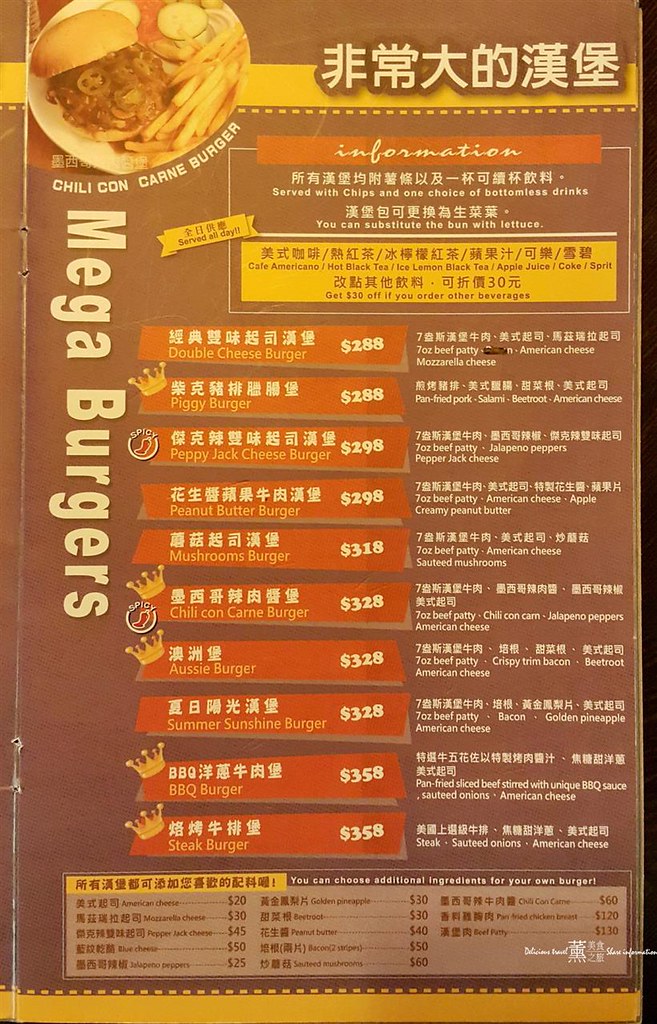This image depicts a page from a Chinese restaurant menu, set against a brown background. Notably, the top-center-right section of the menu features Chinese characters. On the top-left corner, there is a photograph showcasing a white plate carrying a deconstructed burger with brown meat, jalapeños, and components reminiscent of a sloppy joe. This is accompanied by a serving of French fries, along with sliced vegetables including two cucumbers and a tomato, separated as side elements.

Beneath the image, the words "Chili Con Carne Burger" are displayed prominently in white letters. To the left, the term "Mega Burgers" is written vertically, accentuating the headline in a sideways orientation. The main section of the menu lists various food items, elaborately arranged.

Adjacent to the Chinese name at the top right, a red rectangle with white text reads "Information." Below it are Chinese characters, followed by an English translation indicating dishes served with chips and a choice of bottomless drinks. Further down, there's an option to substitute the burger bun with lettuce.

Next, a yellow rectangular box with red font displays Chinese characters, detailing drink options such as Cafe Americano, hot black tea, iced lemon black tea, apple juice, Coke, and Sprite. At the menu's bottom, items are organized within red rectangles. Each rectangle presents a dish's Chinese name in white at the top, its English translation at the bottom, and the price alongside in white within the same red rectangle.

Next to these descriptions, additional details about the dishes are provided in both Chinese and English. The bottom section of the menu features approximately ten items listed in red rectangles running vertically down the page. Concluding the page, a long rectangular box spans the menu width, listing numerous items. This box contains about fifteen different items arranged in three columns, each with their Chinese name, American translation, and price indicated successively.